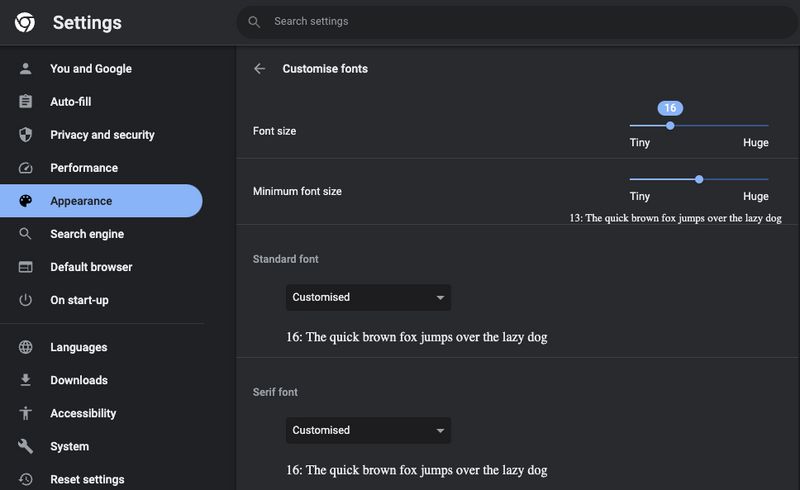The image depicts a settings screen on a computer with a sleek black background. In the upper left corner, a gear icon is accompanied by the word "Settings." To the right of this icon, there is a search bar labeled "Search settings." 

On the left side of the screen, a vertical menu is positioned, listing various configuration options. From top to bottom, the options are: "You and Google," "Autofill," "Privacy and Security," "Performance," "Appearance," "Search engine," "Default browser," "On startup," "Languages," "Downloads," "Accessibility," "System," and "Reset settings." The "Appearance" option is currently highlighted with a blue bar, indicating that it is the selected category.

The right side of the screen displays detailed settings for appearance customization. At the top, it shows "Customize fonts," followed by "Font size" with an adjustable slider ranging from "Tiny" to "Huge." The current setting is a font size of 16, leaning towards the "Tiny" end of the scale. Below this, "Minimum font size" is another adjustable option, also ranging from "Tiny" to "Huge." The chosen minimum font size is set to 13, which is approximately halfway on the scale. A sample text, "The quick brown fox jumps over the lazy dog," is displayed to show the font size in action.

Further down is a section labeled "Standard font," featuring a dropdown menu that says "Customize." The standard font size is set to 16, as indicated next to the sample text "The quick brown fox jumps over the lazy dog." Next, the "Serif font" section is outlined in a similar manner, with a customizable dropdown menu. It also shows a font size of 16 and the sample text "The quick brown fox jumps over the lazy dog."